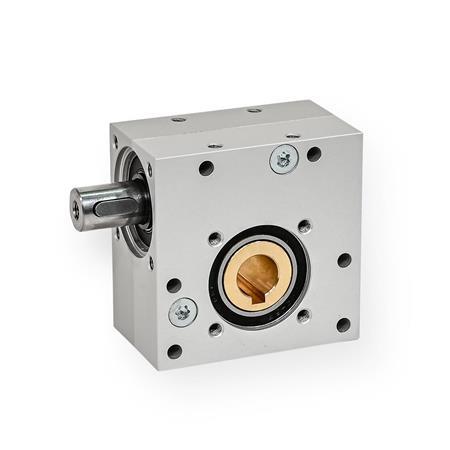The image displays a gray, box-shaped industrial item that appears to function as an adapter or a locking mechanism. The box is predominantly silver or gray, with a cylindrical protrusion on the top left side, resembling a connector or a fuse. This protrusion is surrounded by a circular, possibly metallic, detail. The front face of the box is dotted with several drilled holes, ten to be precise, contributing to the industrial aesthetic. A central feature on the front is a hole with a brass or gold-colored inner circle, which might serve as a locking mechanism. Additionally, there are four drilled holes on the top surface and four more encircling the left side’s protrusion. The central front hole has a distinctive tan or peach-colored backing with a brownish detail, which might be a connector or part of the locking mechanism. The overall appearance suggests it's an industrial component designed to be integrated with other equipment, perhaps as a fuse box or a locking device.